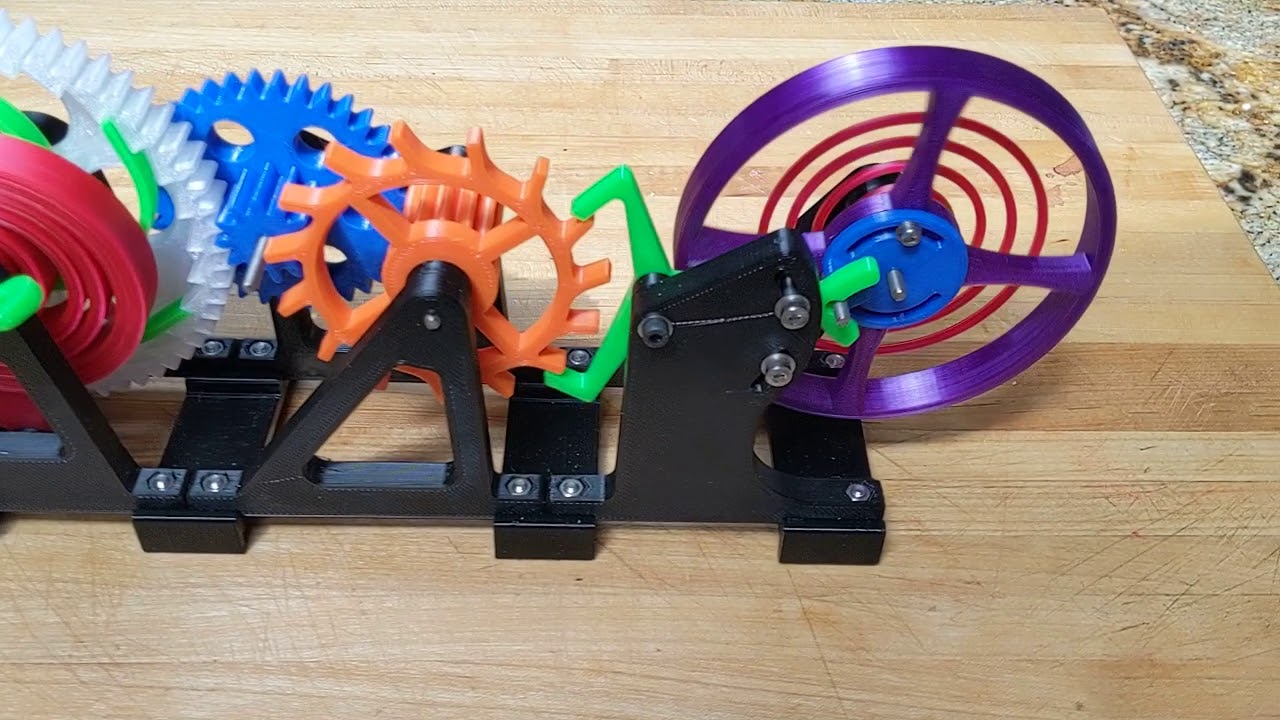This is a photograph of a colorful 3D-printed gear mechanism, likely a toy or educational model, situated on a light wood table or cutting board, adjacent to a marble or Formica countertop in a kitchen setting. The mechanism is built upon a black metal frame and features a series of interconnected gears. The composition includes a red spiral shape, a large white gear, a smaller blue gear, and an orange gear at the center. A green claw connects to the orange gear, enabling a tick-tock motion. On the right, a purple wheel with red interior wheels completes the array. The design suggests a clock-like or wind-up car mechanism, utilizing coils to store and release energy.